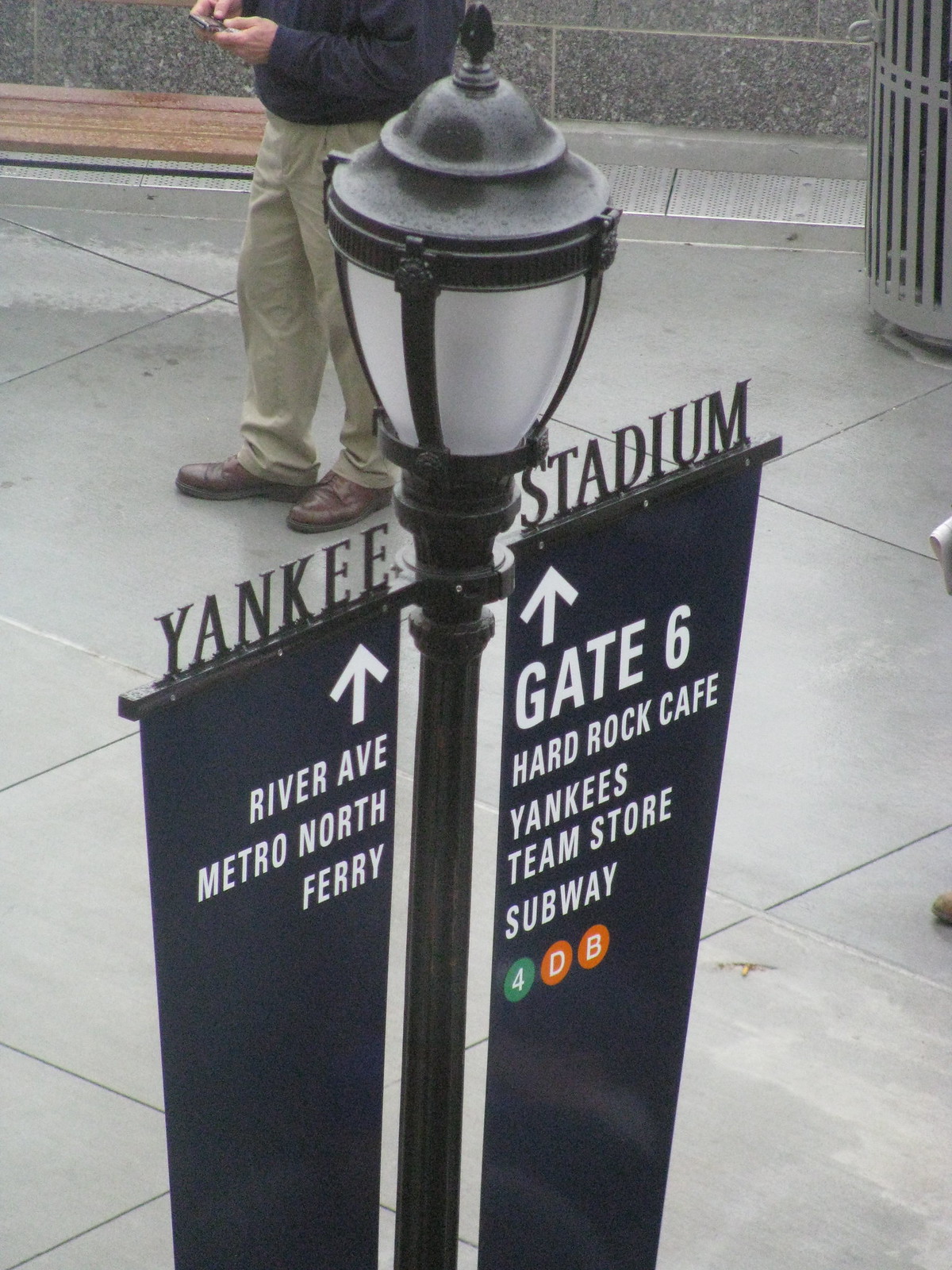This photorealistic image captures a lamppost from a slightly elevated vantage point, revealing detailed elements on and around it. The black lamppost features two metal protrusions near the top, resembling wings that extend horizontally. On these extensions, black, three-dimensional letters spell out "Yankee" on the left and "Stadium" on the right. Each of these protrusions supports a navy flag; the left flag displays a white arrow pointing right with the text "River Avenue, Metro North Ferry," while the right flag shows an upward-pointing white arrow with the text "Gate 6, Hard Rock Cafe, Yankees Team Store, Subway," followed by three circles indicating subway lines—a green circle with the number 4, and two orange circles with the letters D and B.

In the background, the ground is paved with large stone slabs. The lower part of a person is visible at the top of the frame, wearing tan pants, a brown sweater, and brown shoes, engrossed with a cellphone. A garbage can and additional shoes suggest more individuals are present but are partially obscured by the frame. The image provides a dynamic glimpse into the site near Yankee Stadium, complete with navigational signs and a hint of the daily pedestrian activity.